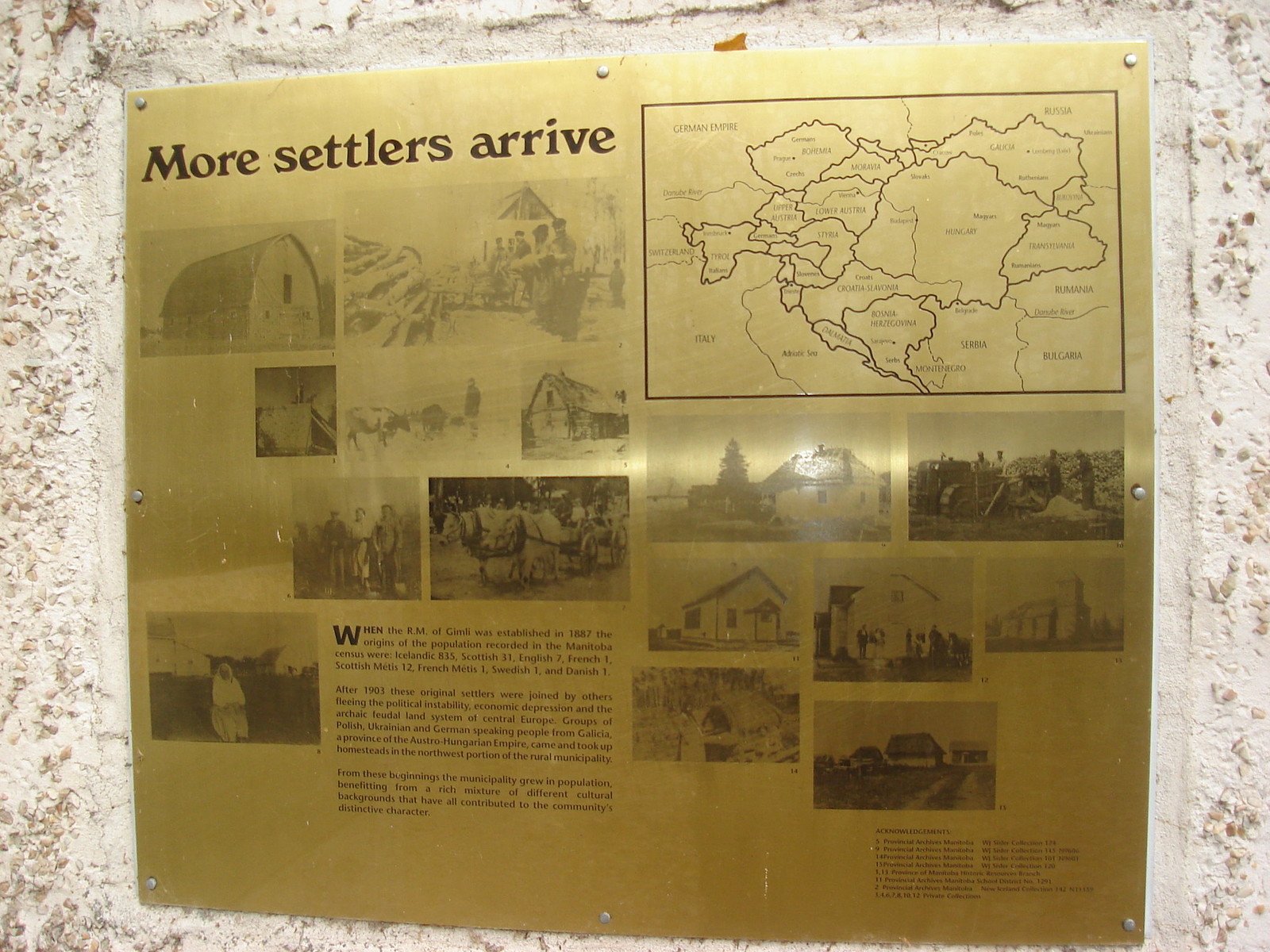The image features a brass sign mounted on a marble wall, which is bordered by light cream and beige stone. The sign, possibly located in a museum, reads "More Settlers Arrive" in engraved dark letters in the upper left corner. To the right of the sign, a portion of a map of Europe is visible, with the specific countries highlighted and outlined distinctly labeled "German Empire."

Below the text, there is a collection of black and white photographs, though they are quite faded and difficult to make out clearly. The images depict various scenes of cabins, farms, settlements, herds of cows, livestock, and some people who likely lived and worked in these areas. These photographs overlay the brass background of the sign.

Underneath the photographs, there is a segment of text, which includes details from a historical record: "When the RM of Gimli was established in 1887, the origins of the population recorded in the Manitoba census were Icelandic 835, Scottish 31, English 7, French 1, Scottish Métis 12, French Métis 1, Swedish 1, and Danish 1."